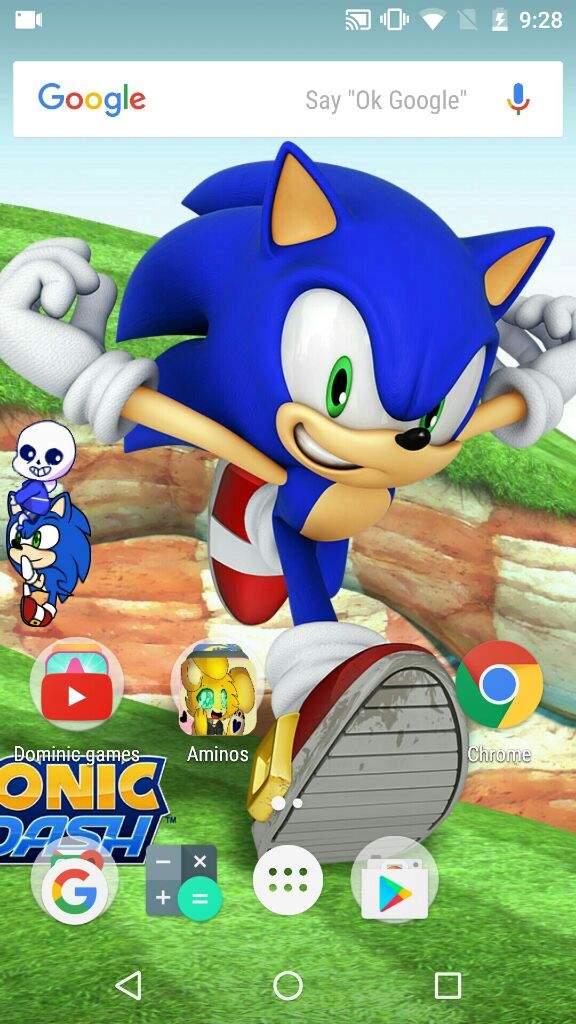This is a detailed photograph showcasing the home screen of an Android phone. The background wallpaper prominently features a dynamic and action-filled image of Sonic the Hedgehog running on a lush grassy field. At the top of the screen, there is a search bar flanked by the Google logo on the left, followed by the text "Say OK Google" in small grey letters, and a microphone icon on the right.

Situated below the search bar, a row of application icons adorn the screen. Starting from the left, there is an icon for "Domino Games," next to it an icon for the game "Aminos." On the right side of Sonic's foot, the familiar Chrome browser icon is clearly visible.

At the bottom of the screen, a dock displays five additional icons. From left to right, these include the Google app, a calculator app icon, an icon represented by an image of a white button akin to a shirt button, and finally, the Google Play Store icon. The alignment of the icons in the first row, "Aminos" and Chrome, aesthetically frames Sonic the Hedgehog's foot, creating a visually pleasing and organized layout.